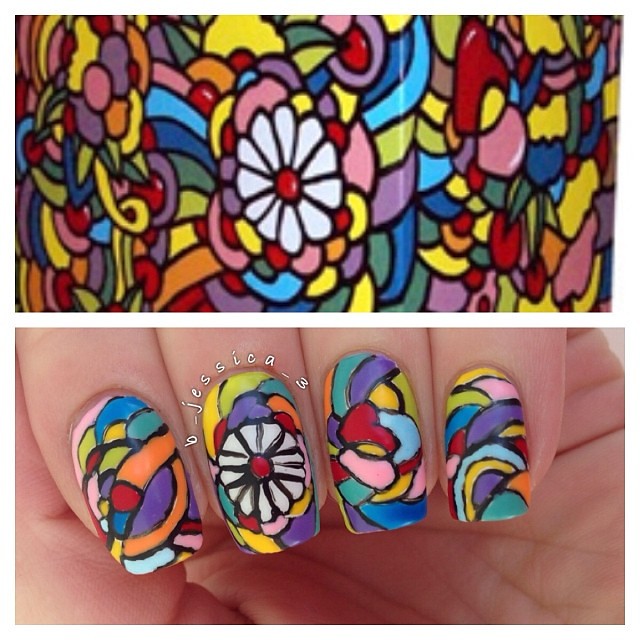The image is a rectangular collage consisting of two sections. The top section is a close-up photograph of intricate nail art showcasing a vibrant and eclectic design. This design features a central white floral pattern surrounded by abstract shapes in a variety of bright colors, including yellow, orange, blue, pink, and red, all outlined in black. There are also globular elements that resemble berries, contributing to the overall floral theme. "Be Jessica 3" is written in white text on one of the nails.

The bottom section of the collage displays four carefully manicured fingers of a female hand, with the same detailed nail art applied. The nails are painted in a multi-color fashion reminiscent of the 1960s Flower Child aesthetic, similar to the stylized chaos of the Sgt. Pepper's Lonely Hearts Club Band album cover. Despite the hand-drawn appearance of the design on the nails, which includes hearts and vibrant hues outlined in black, the artistry mirrors the precision and bright palette seen in the close-up image above.